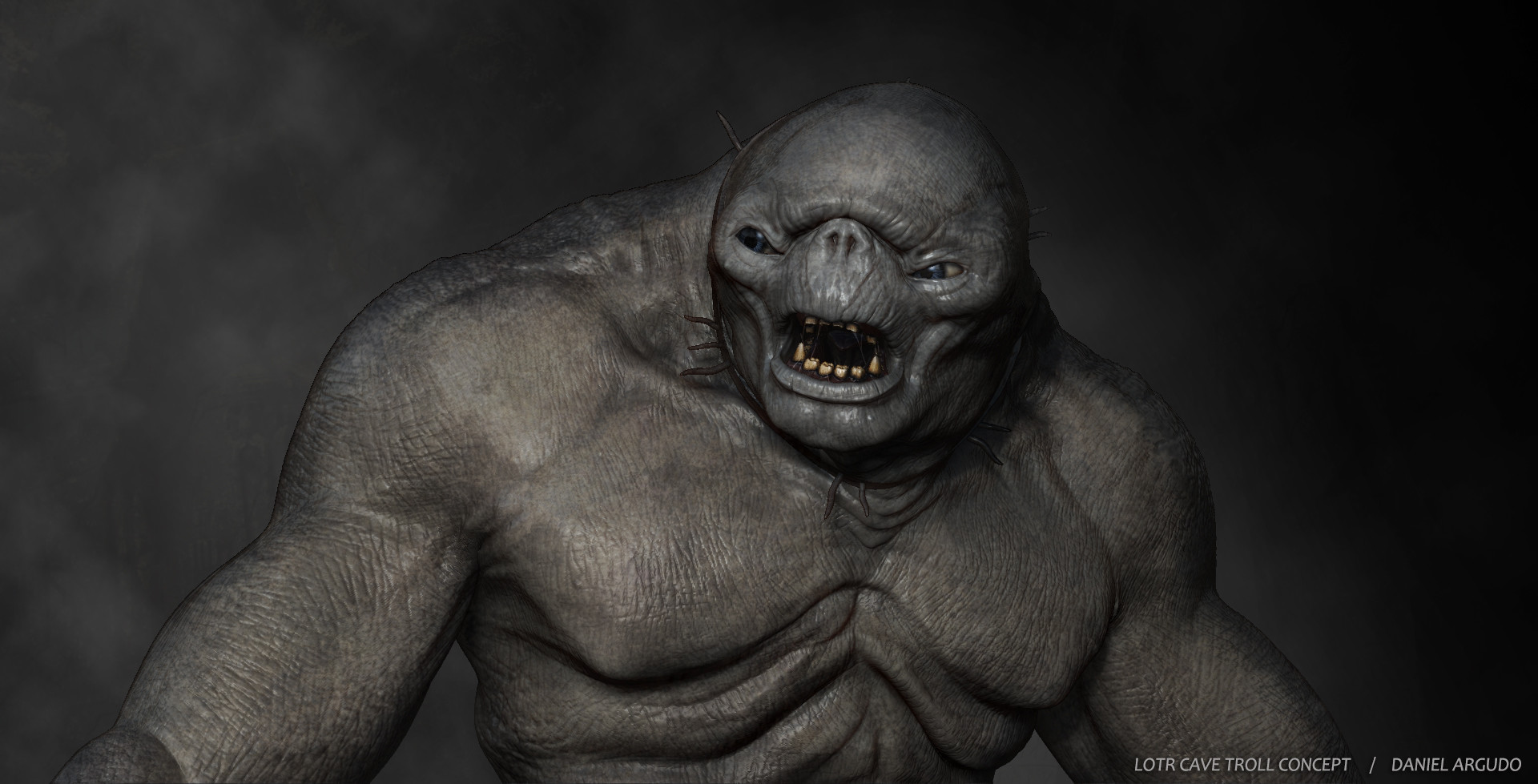This detailed digital rendering, labeled "L-O-T-R Cave Troll Concept by Daniel Argudo" in the bottom right corner, depicts a monstrous cave troll from Lord of the Rings. The troll stands against a muted black and grey gradient background. With no hair or clothing, the troll’s extremely muscular physique is prominently showcased. Its skin, textured like rough elephant hide, is a grayish-brown to navy green hue, adding to its menacing presence.

The troll’s narrow, squinty eyes are set wide apart on the sides of its large, almost neckless head. Its face features sunken cheeks and a distinct, smushed-in nose that sits higher than typical, reminiscent of a bulldog’s. Above the nose is a pronounced wrinkle, further adding to its grotesque appearance. Its mouth gapes open, revealing mostly flat, yellow teeth with two sharper canines and a visible black tongue inside.

The troll’s broad, well-defined shoulders connect directly to its head without a visible neck, enhancing its fearsome look. The chest, depicted from the sternum upward, shows defined muscles converging near the center. Despite its monstrous form, the rendering captures detailed anatomy, giving the troll a terrifyingly realistic touch.